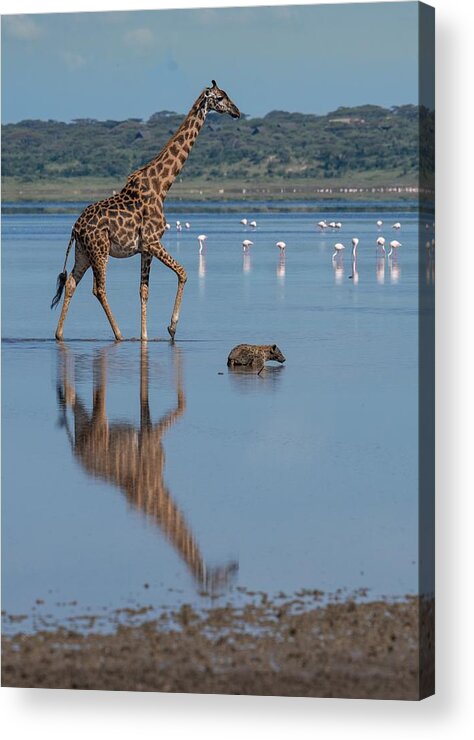In this detailed photograph, the main focus is on a tall giraffe, with its characteristic brown and yellowish pattern, long neck, and long legs, moving gracefully through a shallow body of water, which reflects its majestic form. Alongside the giraffe is a smaller, light brown, four-legged animal that resembles a small hyena or a dog-like creature, also reflected in the water. Scattered throughout the shallow water are numerous white birds, possibly cranes, herons, or flamingos, numbering between 10 to 20. The scene is set against a backdrop of grassy plains and tree-covered hills, with mountains cloaked in green foliage rising in the distance, suggesting the aftermath of heavy rains which have left the dry, grassy plains intertwined with pools of water. The image captures the tranquility and richness of the wildlife in this picturesque landscape.